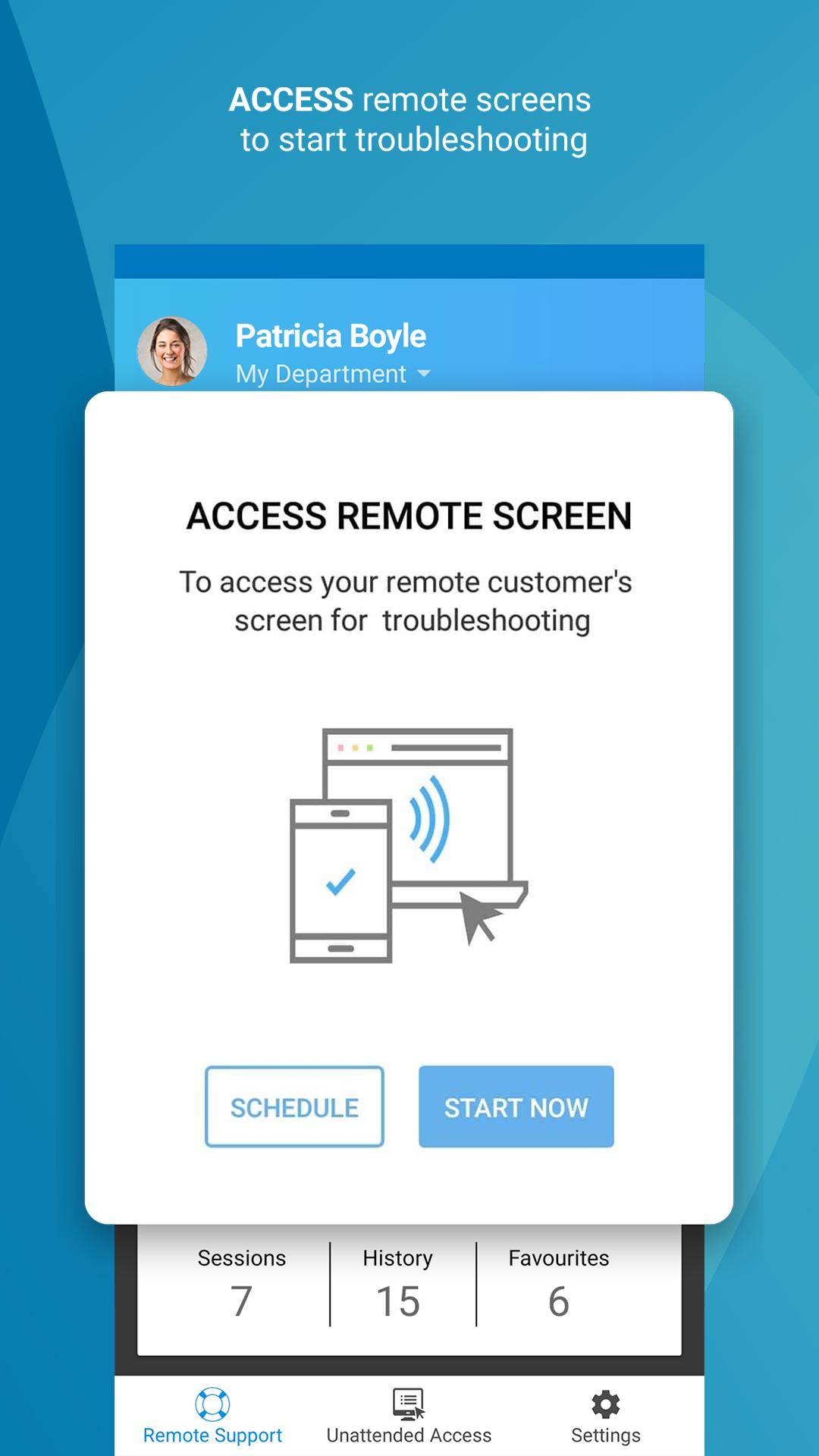The image features a cropped screenshot of an app interface designed for accessing remote help. The background at the top is blue with centered text. In bold white letters, it says "Access," and beneath it, in smaller white letters, it reads "remote screens to start troubleshooting." Below this text, there is a profile picture of a woman. To the right of the profile picture, it says "Patricia Boyle, my department," in small white letters.

In the middle of the screen is a white pop-up. At the top of the pop-up, in bold black letters, it states "Access Remote Screen." Below, in smaller black letters, the text advises, "To access your remote customer screen for troubleshooting." The pop-up also includes a simple line drawing of a laptop and a cell phone.

At the bottom of the screen, on the left side of the pop-up, there is a white button labeled "Schedule." On the right side, a blue button is labeled "Start Now."